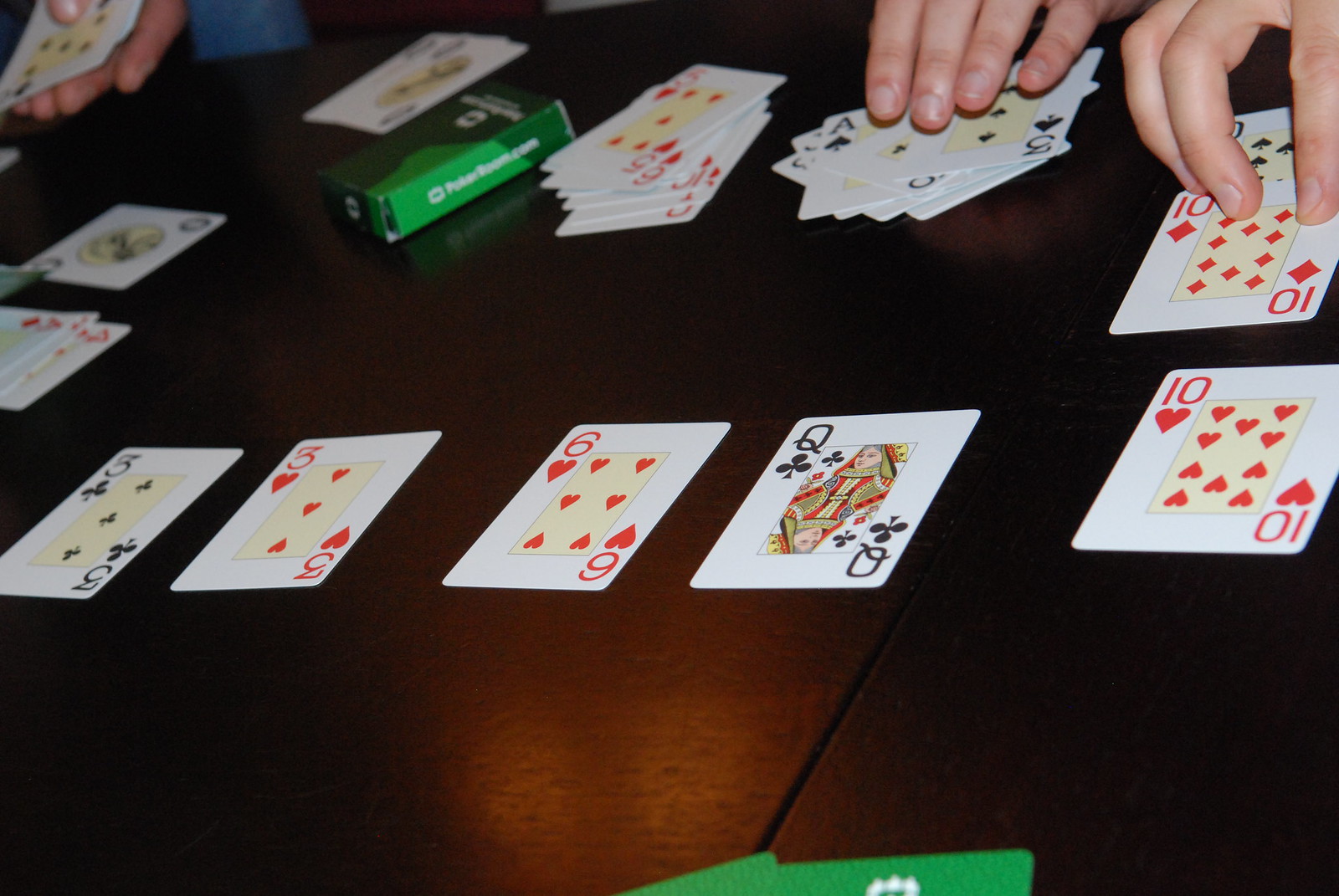This image captures an intense moment of a card game among several people. In the top half of the frame, three different hands are engaged in play, with a wooden table serving as the backdrop. The playing cards in sharp focus include a black Three of Clubs, a red Three of Hearts, a red Six of Hearts, a black Queen of Clubs, and a red Ten of Hearts. A stack of cards is visible next to the players' hands. In the background, a green box can be seen, though its purpose is unclear—it could either be a card box or something else entirely. Additionally, in the lower right-hand corner, there is a glimpse of what seems to be the top of some green cards. The polished surface of the wooden table catches the light, casting a subtle reflection that adds to the atmosphere of the scene.